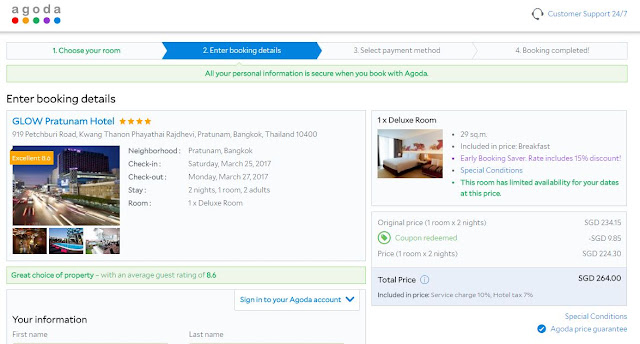Sure, here's a detailed and cleaned-up caption for the image:

---

The top left corner features the brand name "Accorda" written in grey, with colored circles below each letter: red under 'A', orange under 'C', green under 'C', purple under 'O', and blue under 'R', 'D', and 'A'. To the top right, "Customer Support 24x7" is displayed in blue text.

Below the brand name, on the left side, a step-by-step booking process is outlined: "Choose Your Room" (Step 1, in green, indicating completion), "Enter Booking Details" (Step 2, highlighted in blue), "Select Payment Method," and "Booking Completed" (both grey). Under these steps, a green text notes, "All personal information is secure when you book with Accorda."

Further down, on the left, in blue text, it prompts to "Enter Booking Details" for "Glow, Pratunam Hotel," rated 4 stars (stars in yellow). The address is given as "919 Pechburi Road, Kwangtunan, Payatai, Rajhevi, Pratunam, Bangkok, Thailand, 10400, Neighbourhood Pratunam, Bangkok." 

The check-in date is Saturday, March 25, 2017, and check-out is Monday, March 27, 2017, with a 2-night stay in 1 deluxe room for 2 adults. At the bottom, a green text states, "Great choice of property with an average rating of 8.6."

Toward the bottom left, text in blue urges users to "Sign in to your Accorda account."

On the right side, the reservation details are more specific: "1x Deluxe Room, 29 square meters, includes breakfast," and mentions an "Early Booking Save Rate" with a 15% discount, in purple. "Special Condition" is highlighted in blue, indicating limited availability for the chosen dates (text in green).

At the very bottom, the pricing breakdown is detailed: the original price for 1 room for 2 nights is SGD 234.15, with a green "Coupon Redeemed" reducing the price by SGD 9.85. The final price is SGD 224.30, with a total price of SGD 264.00 including all fees. "Special Condition" and "Accorda Price Guarantee" are highlighted in both green and blue.

---